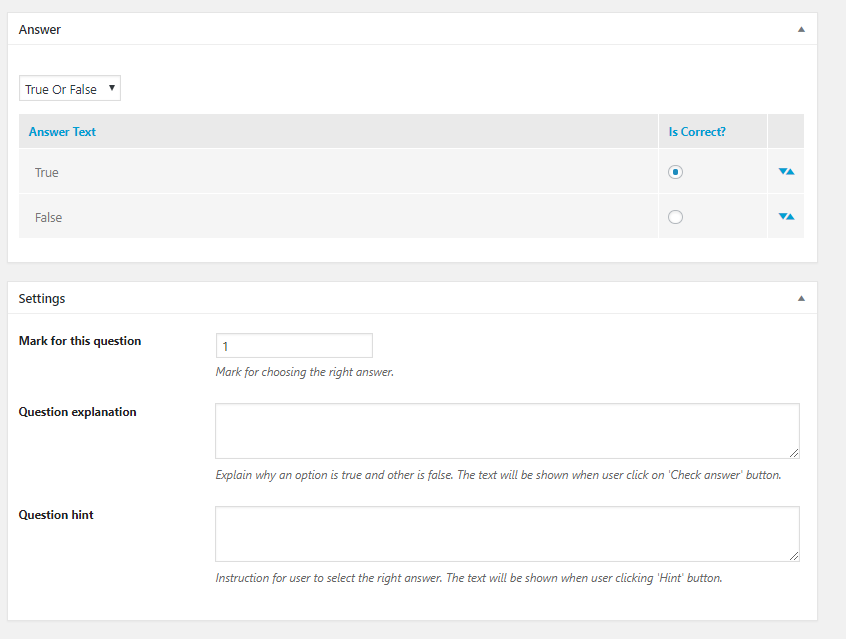This image is a screenshot of a website’s quiz settings interface. At the top left, the interface has a section labeled as “Answer” which appears to be configured for creating a question. The "Answer" section allows selection of answer types from a drop-down menu, with the current selection being "True or False." 

Beneath this, there are fields labeled "Answer Text" with the options "True" and "False," where "True" has been selected, indicating it is the correct answer for the unseen question.

Further down, there is a “Mark” section indicating that correctly answering this question will yield one point. It also includes a "Question Explanation" field where users can provide reasons or explanations for the correct answer. 

At the very bottom, there's a “Question Hint” option, designed to offer hints to users who may need assistance in answering the question. This setup suggests a comprehensive and user-friendly interface for designing interactive quizzes or assessments.